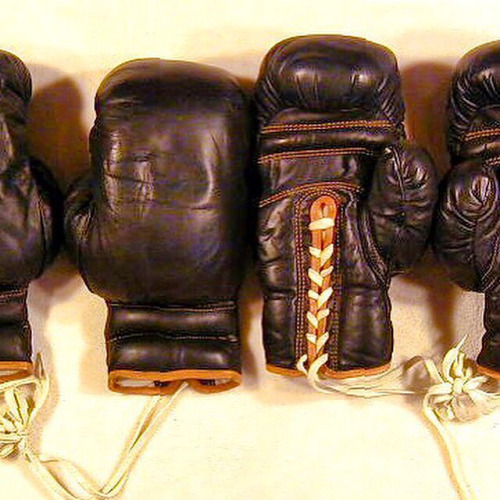This image features an array of four vintage brown leather boxing gloves arranged against a backdrop that varies between brown, tan, yellow, and peachish white shades, adding to its aged appearance. Each glove, predominantly dark brown, is detailed with orange stitching and trims around the palm and wrist area, showcasing intricate craftsmanship. The laces, primarily white or light-colored, elegantly dangle from the gloves. 

On the far left, a partial view of a glove reveals just the edge of the thumb and opening. Adjacent to it on the right, another glove sits thumb-side out, its entire form more visible. In the center, one glove faces palm up while its counterpart is palm down, highlighting the orange stitching that runs across the palm area and the white laces intricately woven through. On the extreme right, only the base and thumb of the final glove are partially visible. Shadows cast by the gloves on the surface below enhance the image's depth and nostalgic feel, reminiscent of an old, carefully preserved photograph.